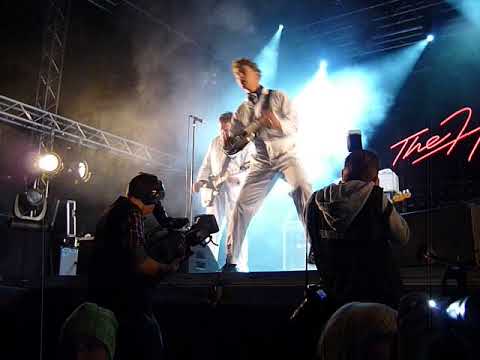In this detailed concert image, a dynamic scene unfolds with multiple focal points. Dominating the center, a man dressed in all white stands on a well-lit stage, playing a guitar and surrounded by intricate lighting arrangements and silver trusses. Above him, a black banner with partially visible, red cursive script hints at the name "JES." The backdrop is characterized by a variety of vivid colors, including white, red, black, gray, blue, and silver, accentuated by circular white lights.

In the lower right corner, a young Caucasian man, identifiable by his gray baseball cap and yellow earplugs, aims a camera towards the stage, capturing the performance. He is among several other photographers and videographers, indicating the importance of documenting this indoor concert. The venue features black tarp-like walls, adding to the intimate, focused ambiance of the event. Crisscrossing beams and structures further frame the concert setting, reinforcing the technical sophistication behind the performance.